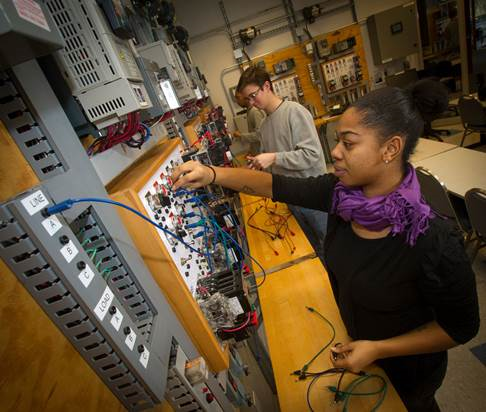In an educational or instructional setting focused on electronics, a black woman with dark hair neatly tied up in a bun is seen wearing a black shirt and a purple scarf around her neck. She is actively engaged with an electronic switchboard mounted on the wall in front of her, her right hand adjusting a knob while her left hand holds green and blue cables, connecting them to the board. Visible on her right forearm is a tattoo, and she has a bracelet on her wrist. The switchboard displays various labeled terminals, including "line ABC" and "load ABC," and is surrounded by blue and green cables. To her left, slightly behind her, stands a Caucasian man with short cropped brown hair, wearing glasses, a gray sweatshirt, and jeans. He is also focused on another segment of the switchboard. In the background, there is another person partially visible, with dark hair and wearing a green sweater. The room contains a white table with metal chairs pushed in, and similar switchboards and electronics mounted on the walls and plywood, contributing to the classroom environment.